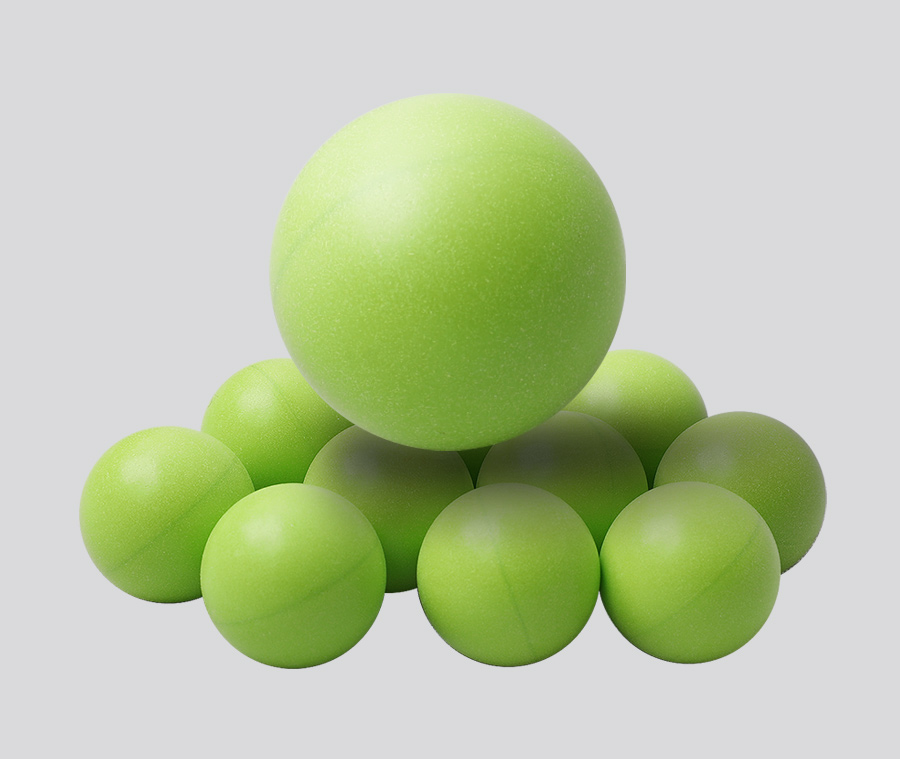The image depicts a digital illustration of various green balls arranged against a completely white background. The composition features a layer of nine smaller balls, all clustered together, each exhibiting a light, bright green color reminiscent of a golden lime. Midway around each smaller ball is a thin seam in a darker shade of green. Situated atop this cluster is one significantly larger, identical green ball, which is about four times the size of the smaller ones. This larger ball shares the same light green hue and possesses a matching seam. The balls exhibit subtle shading, with light primarily hitting them from the upper left corner, casting gentle shadows towards the lower right.